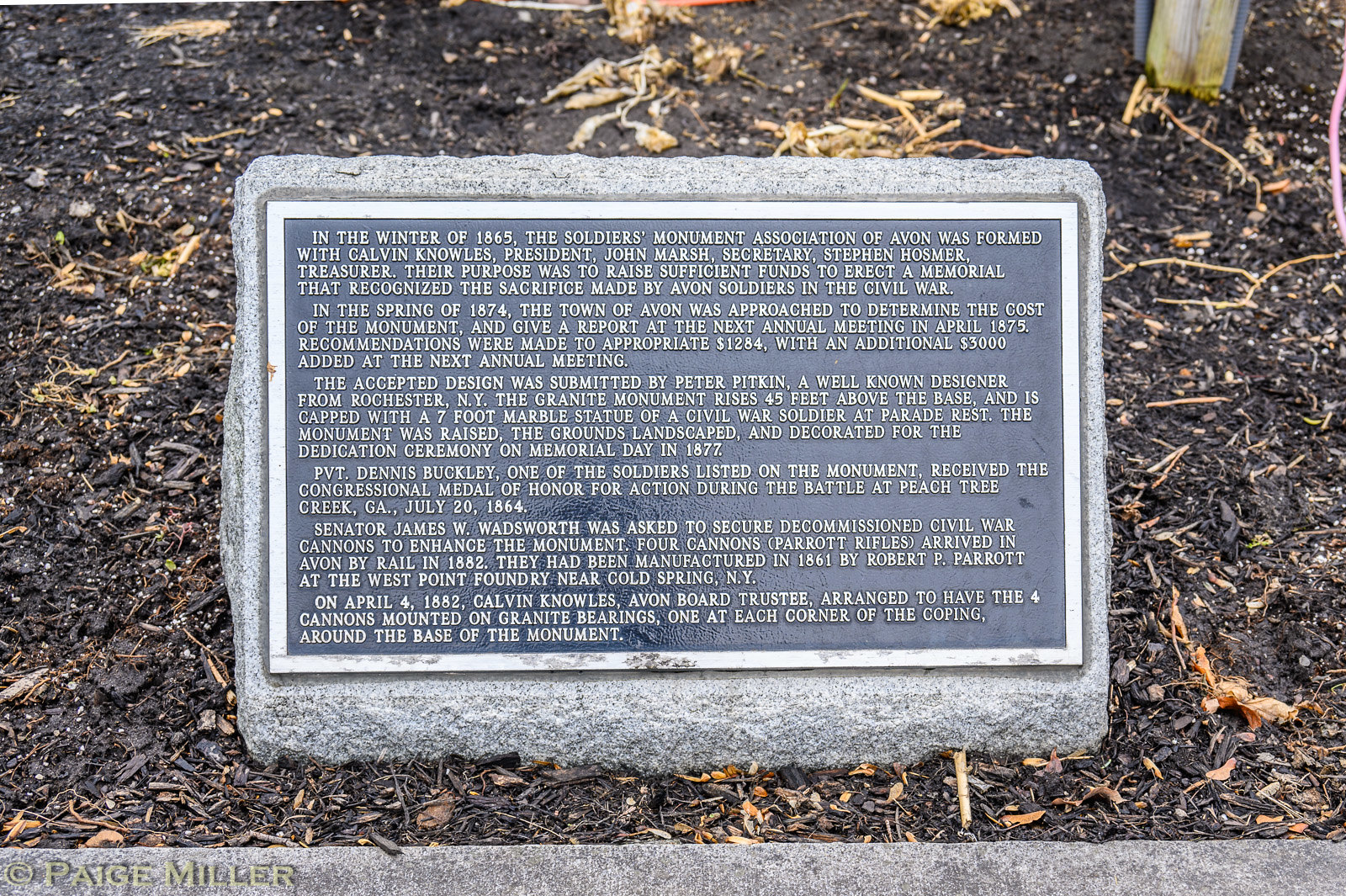The image depicts a historical marker dedicated to the Soldiers' Monument Association of Avon, prominently featuring a black plaque with silver text set atop a granite stone, angled forward for easy reading by passersby. The plaque is situated in a dark soil area, resembling a garden setting. The inscription begins: "In the winter of 1865, the Soldiers' Monument Association of Avon was formed with Calvin Knowles, President; John Marsh, Secretary; and Stephen Hosmer, Treasurer." Their goal was to raise funds for a memorial honoring the sacrifices of Avon soldiers in the Civil War. By the spring of 1874, the town of Avon evaluated the monument's costs, ultimately recommending an initial appropriation of $1,284, supplemented by $3,000 the following year. Designed by Peter Pitkin from Rochester, New York, the 45-foot granite monument features a 7-foot marble statue of a Civil War soldier at its peak. Dedicated on Memorial Day in 1877, the monument's grounds were beautifully landscaped for the occasion. Notably, PVT Dennis Buckley, a soldier commemorated on the monument, received the Congressional Medal of Honor for his actions at Peach Tree Creek, Georgia, on July 20, 1864. Upon Senator James W. Wadsworth's efforts, four decommissioned Civil War cannons arrived in 1882, manufactured in 1861 by Robert P. Parrot at the West Point Foundry. These cannons were mounted on granite bearings at each corner of the monument's base by Calvin Knowles, an Avon board trustee. The plaque includes a watermark of the photographer, Page Miller, on the bottom left, indicating their attribution.